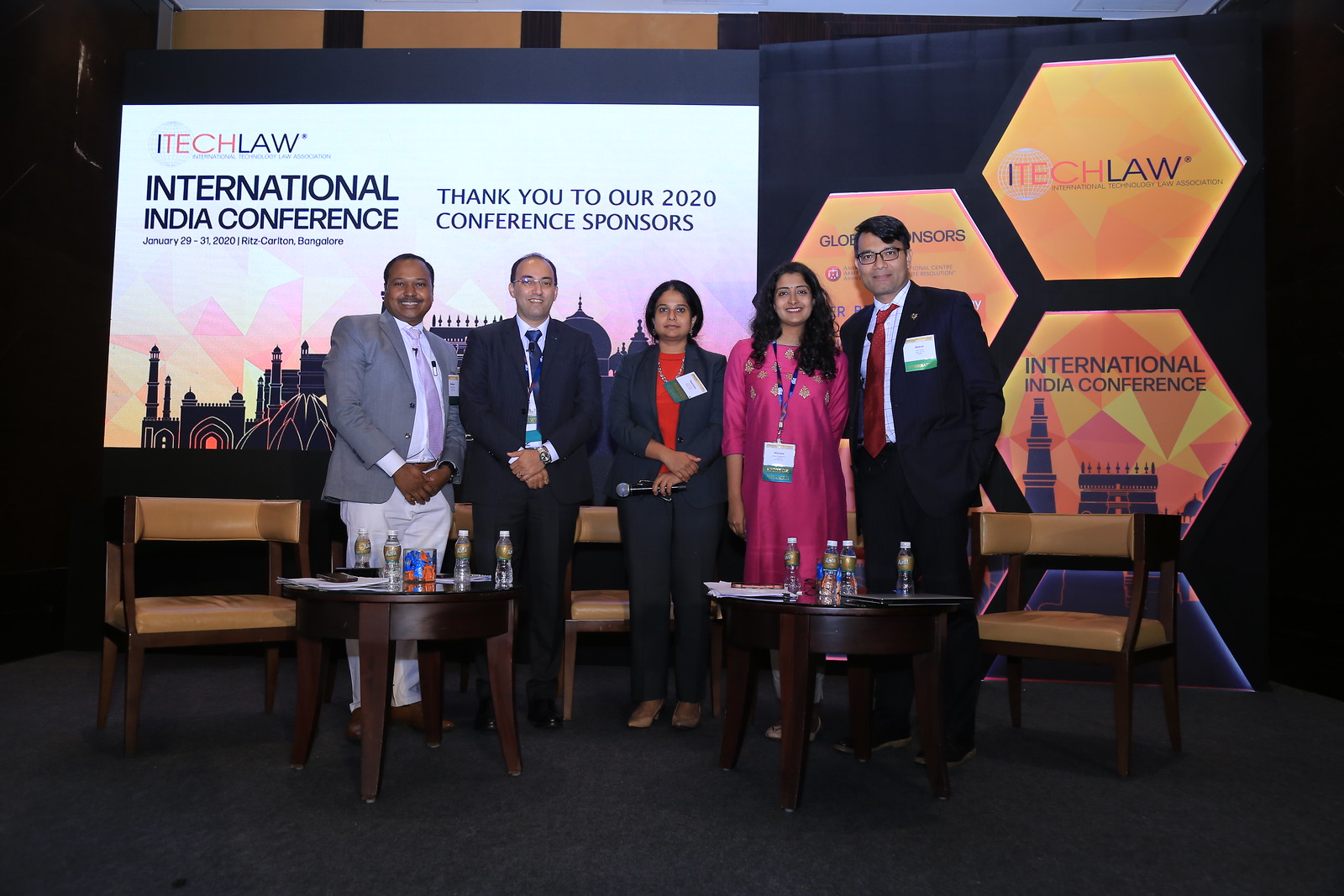The image captures a moment from the I-Tech Law International India Conference held from January 29th to 31st, 2020, at the Ritz-Carlton in Bangalore. Five individuals of Indian heritage are standing on a stage or platform, dressed in formal business attire. From left to right, a man in a gray jacket with a buttoned front stands with his hands folded, followed by another man in a dark suit and glasses. In the center, a woman with short black hair, dressed in a gray suit and holding a microphone, gazes forward with a solemn expression. Next to her is a woman with long black curly hair, wearing a vibrant pink-purple dress, and finally, a tall man in a black suit with a red tie and glasses stands on the far right. The backdrop behind them is a black wall adorned with a white poster that reads "International India Conference" with the I-Tech Law logo and conference details. Yellow and orange hexagonal shapes with text are also visible. In front of the group are two small round brown tables with water bottles. The scene is set with beige wooden chairs and additional text thanking the 2020 conference sponsors. The photo embodies a formal and professional atmosphere, capturing a significant moment at the conference.